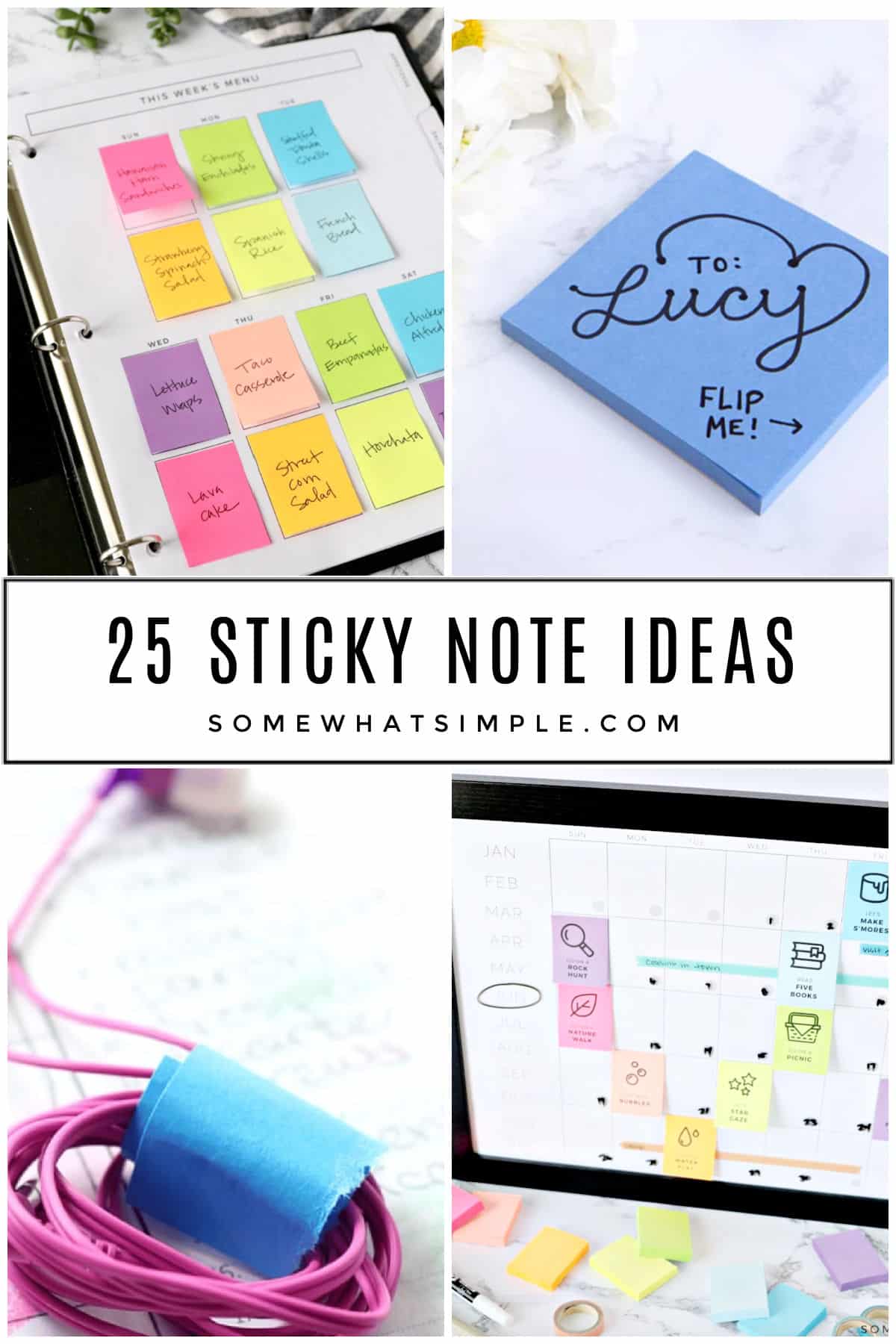The image is a collage divided into four quadrants, with a central label that reads "25 Sticky Note Ideas" and the web address "SomewhatSimple.com," written in black on a white background. Each quadrant creatively showcases various uses for sticky notes. The top left quadrant features a planner open to a weekly menu; each day is marked with colorful sticky notes listing meals such as lettuce wraps, lava cakes, and taco casserole. The top right quadrant displays a blue sticky note pad with a handwritten message in cursive saying, "To Lucy: flip me," accompanied by an arrow. The bottom left quadrant shows a pair of pink headphones neatly bundled using a blue sticky note as a makeshift cable tie. Lastly, the bottom right quadrant illustrates a computer screen set to a monthly calendar view for June, adorned with digital sticky notes marking a variety of events and reminders like picnics and book-related activities. The overall color palette features light, pastel tones, emphasizing a calm, organized aesthetic tailored for a broad audience.